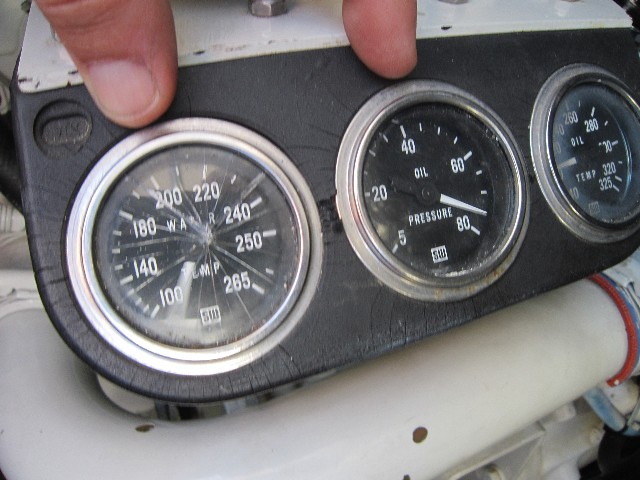This image showcases a horizontal photograph of an unidentified mechanical system, featuring prominently three circular gauges, set within a casing of cracked black rubber or plastic. Thick white PVC piping runs along the bottom edge of the machinery. A hand appears in the frame, with only the thumb (from the bottom knuckle to the nail) and the tip of the index finger visible, poised above two of the gauges.

The leftmost gauge displays numerical markings ranging from 100 to 265, at intervals including 100, 140, 180, 200, 220, 240, 250, and 265. The bottom of this gauge is labeled "SW," and its cracked crystal face reveals additional, unclear lettering. The central gauge is labeled "Oil Pressure," with readings marked at increments of 5, 20, 40, 60, and 80. The rightmost gauge, marked "Oil Temp," shows legible numbers ranging from 260 to 325, with full visibility of 260, 280, 300, 320, and 325.

Due to the angle of the photograph, the detailed context of whether this system is part of a pump, engine, vehicle, or another type of machinery remains unknown.